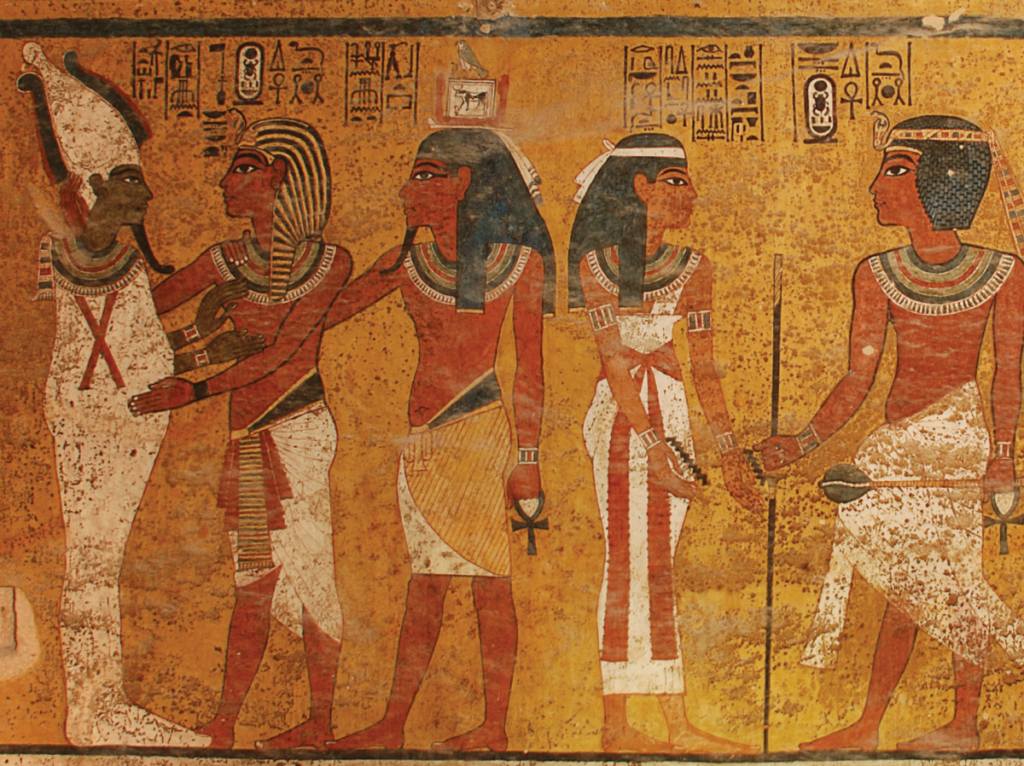This image depicts an ancient Egyptian scene on a yellowish-brown background filled with intricate hieroglyphs. At the top, a gray line runs across, separating the background from the hieroglyphs, which are predominantly black, with some central colored symbols in red, white, and gray. 

The left side of the image features a dark-skinned man adorned in a white hat and robe, who appears to be placing his hands on the chest of another man. This second figure is dressed similarly to the Sphinx, with a striped headpiece and a lower garment. He has no shirt and is being embraced by yet another man behind him, who also sports a minimal robe and has dark skin. 

Further to the right stands a woman in a striking red and white dress, adorned with a green, red, and black collar, and a white ribbon around her dark brown hair. Facing her on the far right is a man in a white robe, holding a sepulcher in his left hand. He appears to be extending his hand towards her, smiling, indicating some form of interaction or possibly a relationship. The backdrop of hieroglyphs and the detailed depiction of the individuals in traditional attire highlight the rich cultural and historical significance of the scene.